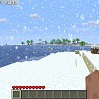This detailed drawing captures a serene winter scene. Snow softly blankets the foreground, creating a pristine layer of white. To the right, a gray wall extends along the side, partially adorned with red objects, adding a touch of color to the monochrome palette. Flakes of snow are gently falling, enhancing the wintry atmosphere. Beyond the snow-covered ground, tranquil blue water stretches across the middle of the image. In the distant background, an island with lush green trees offers a vibrant contrast to the wintry setting. Above, the sky remains a clear blue, dotted with a few clouds, harmonizing the scene with a gentle blend of colors. The compactness of the drawing necessitates close inspection to appreciate its nuanced details.